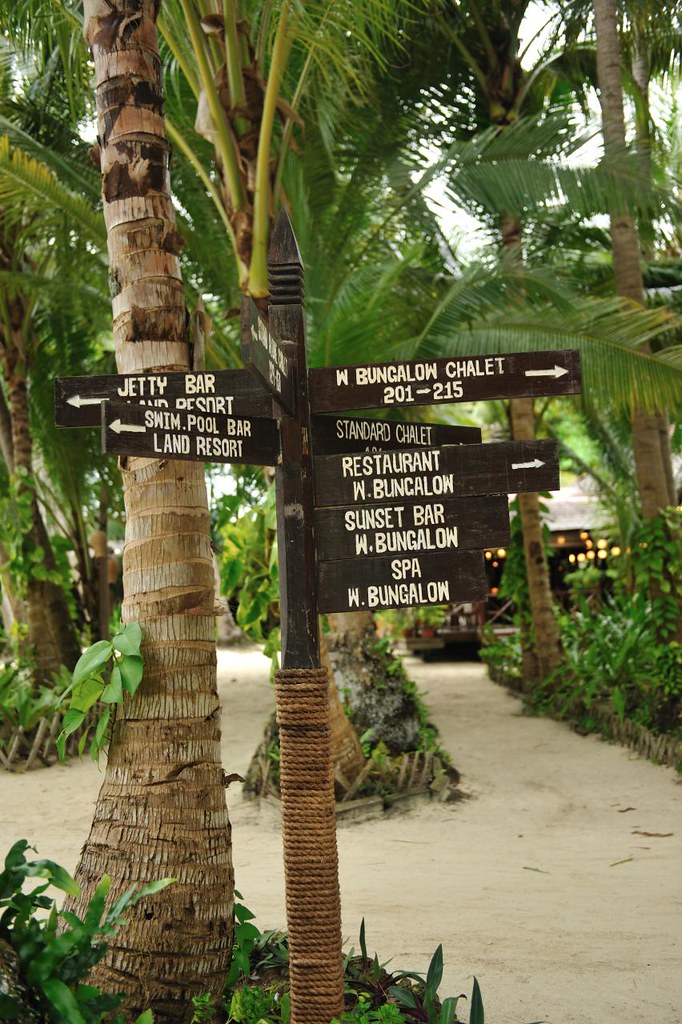The image depicts an outdoor scene at a beach resort on a cloudy day, featuring a sandy walkway lined with well-maintained palm trees and some grassy plants at the base of the trees. Central to the scene is a pole with directional signs pointing to various resort locations. To the left, signs indicate "Jetty Bar and Resort," and "Swimming Pool Bar Land Resort" with arrows pointing leftward. To the right, numerous signs guide visitors to "West Bungalow Chalet 201-215," "Standard Chalet," "Restaurant," "Sunset Bar," and "Spa," all within West Bungalow. In the background, there is a clearly visible building with windows and a brown roof, potentially an outdoor bar. The scene is verdant, orderly, and suggests a welcoming and well-organized resort environment.